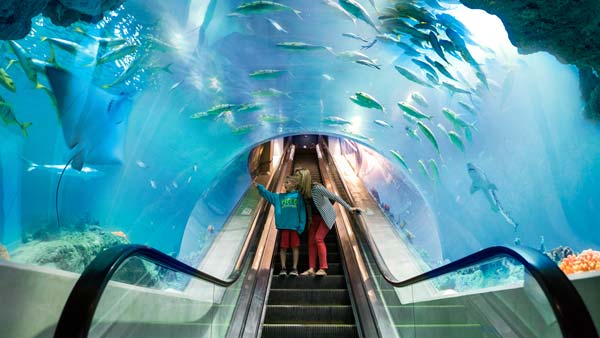Inside a grand aquarium, a captivating scene unfolds as an escalator descends through a tunnel enveloped by a massive, transparent aquatic enclosure. The clear blue water is teeming with marine life, including various green-hued fish, a stingray on the left, and sharks on the right. Emerging from the escalator are a small boy wearing red shorts, a blue long-sleeve sweatshirt, and sneakers, alongside an adult, possibly his mother, dressed in red pants, a blue sweater, and sandals. The child is pointing excitedly at the fish, with both of them gazing in wonder at the vibrant aquatic world surrounding them. The arching aquarium frames their descent, showcasing schools of fish swimming together at the top center, larger fish on the sides, and rich plant life and rocks at the bottom, creating an enchanting underwater vista. They face to the left, engrossed in the mesmerizing display of marine life that stretches above and around them, enhancing the surreal experience of being in a tunnel-like passage within the aquarium.